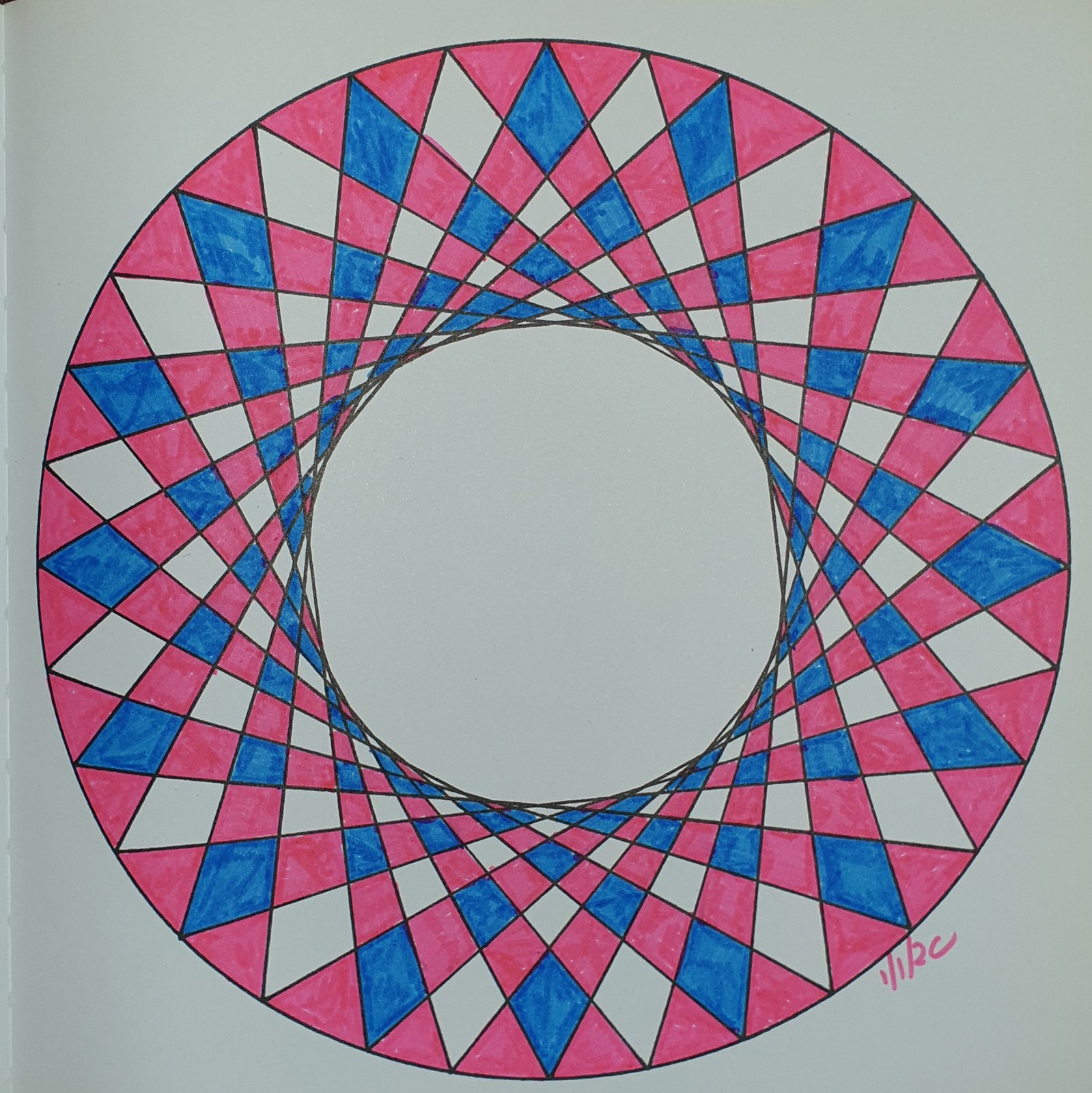The image features a meticulously hand-drawn spirograph design, rendered in black pen. Intricate geometric shapes intertwine to form a captivating circular pattern. The design is further enhanced with delicate splashes of pink and blue watercolor, adding depth and vibrancy. Centered within the spirograph is an inscription, possibly reading "112C," "11BC," or "PC," written in pink. The spirograph's geometric intricacies evoke images of diamonds or checkerboard patterns, depending on one's perspective.